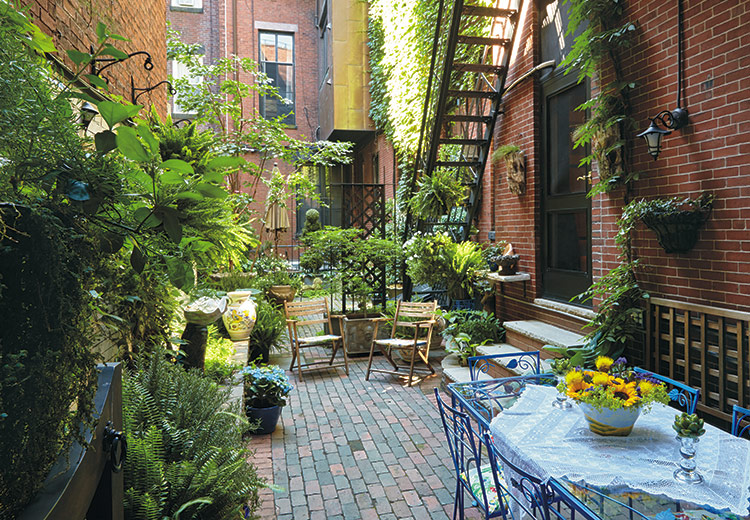A photograph depicts a charming rear terrace of a typical New York-style brick apartment building. The scene is framed by red brick buildings, with the primary building on the right showcasing wrought iron fire escape stairs leading to the second floor. The building's brick wall is adorned with planters, cascading ivy trailing down to the ground, demonstrating a resident's love for greenery. The rear entry door, slightly ajar and stained black, leads to a brick-covered terrace area. The left side of the terrace features a lush wall garden, overflowing with green growth from wrought iron plant hooks mounted on the opposite building wall.

In the foreground, to the right, there is an elegant glass table with five glass chairs, topped with a white cloth and a vase of sunflowers, adding a splash of vibrant color. The setup suggests a peaceful space for outdoor dining. Further back, two brown wooden chairs and various potted plants complete the cozy garden scene. Behind the fire escape, more greenery flourishes, providing a soft, natural contrast to the urban setting. The terrace is an oasis amidst the dense, historic architecture, with another brick building visible in the distance, unconnected to the main structure. This beautifully curated garden terrace captures a serene and lush retreat in the heart of the city.